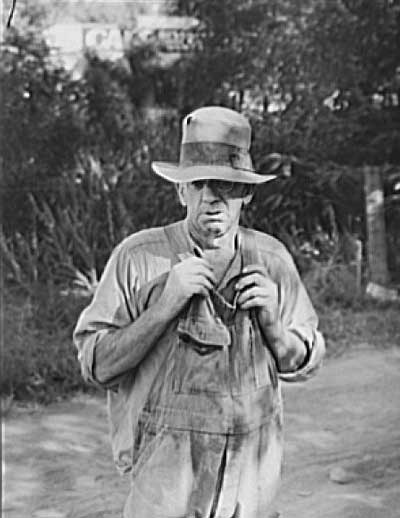In this black and white photograph likely taken in the 1930s, an elderly man stands posing directly towards the camera on a dirt road. He appears to be in his mid to late 60s, wearing heavily worn overalls and a long-sleeve shirt with the sleeves rolled up to his elbows. The overalls are faded, and he grasps the straps with both hands. The man is also wearing a farmer's hat with a cylindrical top and a black, worn headband; the brim of the hat casts a shadow over his face, obscuring his eyes. Round, gold wire-rimmed glasses rest on his nose. Behind him, the dirt road is bordered by a section of grassy field, followed by larger bushes and dense vegetation. This vegetation appears to be a mixture of trees and bushes with thick leaves. There may also be a building obscured by the dense foliage. The man's serene yet authoritative presence and the rustic landscape create a nostalgic snapshot of rural life from a bygone era.